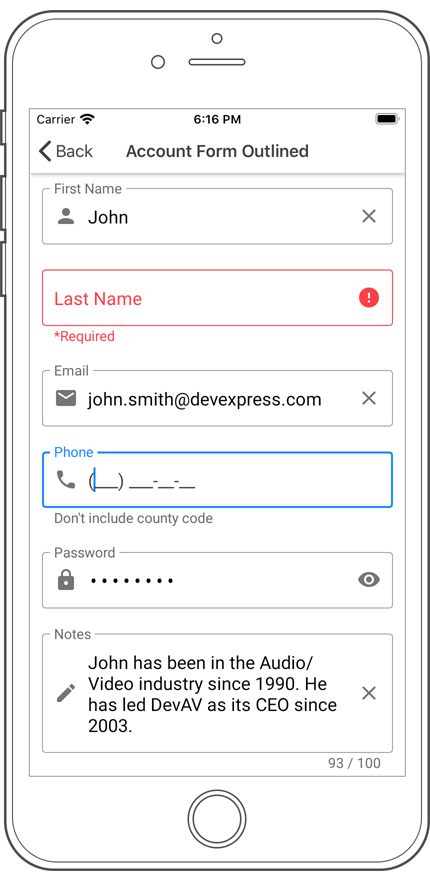The image appears to be a screenshot or digital rendering of a smartphone display, specifically resembling an iPhone due to its rounded edges and prominent circular home button at the bottom. The outer edges of the phone are fully visible, and it features physical buttons on the right-hand side — one smaller button at the top and two larger buttons below it.

At the top center of the screen, a lined speaker area is flanked by two small circles, one on the left and one above the speaker. The interface shown on the screen includes a central boxed area displaying the time "6:16 PM." To the left of this boxed area is a "Back" button with a leftward-pointing arrow indicator.

Below this header is a form layout delineated with several fields. The first section, labeled "First Name," contains a rectangular text box with the entry "John," and an "X" icon on the right side permitting the clearing of the text. The next section, "Last Name," features an orange-outlined text box with a caution icon on the right, although the specific last name entry is not visible.

Underneath the "Last Name" field is a section labeled "Email," which contains a rectangular box displaying the email address "mr.smith@devexpress.com." The "Phone" section follows next, with a blue-outlined rectangular box for entering a phone number. Below the "Phone" entry is a "Password" field, which shows a series of dots to represent hidden characters and a lock icon beside it. 

At the bottom of the form is a "Notes" area containing some pre-written information, along with an editable icon to the right, indicating that this section can be modified.